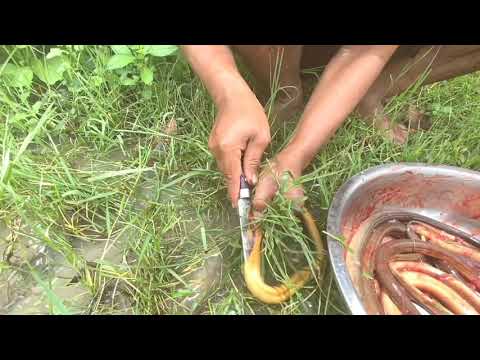In this outdoor image, a person with darker, possibly olive-toned skin is squatting barefoot in a field of sparse green grass and muddy, greenish water. With a red wooden-handled knife in their right hand, they are actively cutting or skinning a yellow eel or snake, which they hold down near the center of the image. Only their lower arms, legs, and bare feet are visible. To the right of the person, there is a metal bowl partially filled with blood and containing several yellow and brown snakes or eels, suggesting that more creatures have already been processed. The scene is set under natural daylight, with no additional text or items in the background.